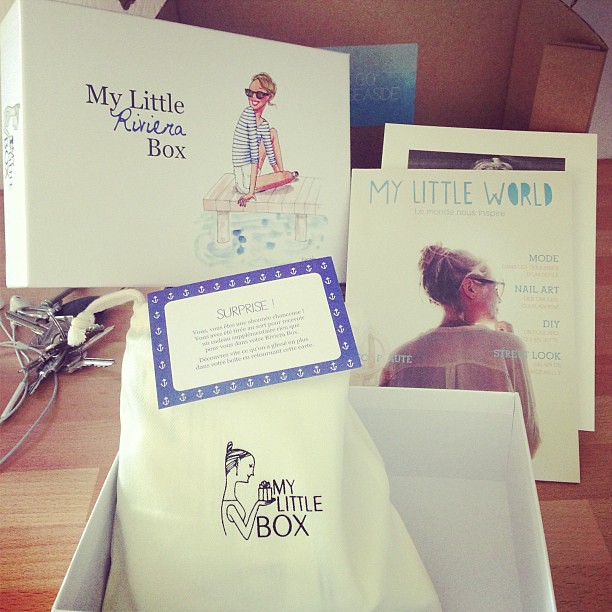The image depicts an opened woman's gift box set on a brown table. The top-left corner features a white box with "My Little Riviera Box" inscribed in elegant scroll, accompanied by an illustration of a woman in a white and blue striped shirt and white shorts, wearing sunglasses, and either standing or sitting on a dock over water. Below and to the right of this box, there's a magazine titled "My Little World," adorned with various article headings such as "Mode," "Nail Art," and "DIY." The magazine cover displays the profile of a woman with her hair up in a bun, wearing glasses, and gazing to her right. 

Central to the composition is a white tote bag, also inscribed with "My Little Box" and featuring a drawing of a woman holding a box. Above this drawing is a white card bordered in blue with anchor motifs, labeled "Surprise," although the text below is illegible. Peeking from behind the magazine is a black-and-white photograph in a white frame, though its details are indistinguishable. Adjacent to the main box, a glimpse of potential car keys is visible on the left-hand side of the table. The scene is meticulously arranged, highlighting the harmonious blend of boxed items and thematic designs.